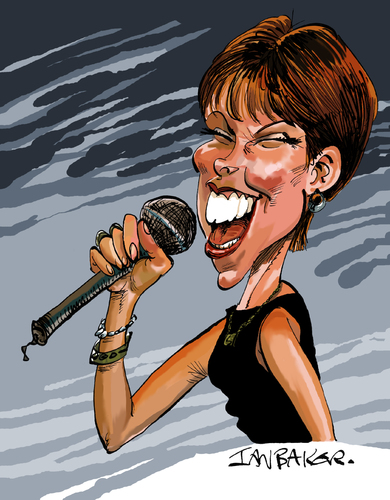In the image, there is a caricature of a redheaded lady singing passionately into a microphone. This digital or poorly-scanned illustration, created by Ian Baker, exaggerates her facial features, giving her a large mouth with big white buck teeth and a smaller nose. Her eyes are closed as she belts out a tune, creating the impression that she might be a terrible singer. The singer, who appears to be in good shape, is depicted wearing a black sleeveless dress along with two bracelets on her microphone-holding right arm - one resembling pearls and the other a green band. She also has earrings and a necklace. The background gradients from dark blue at the top to lighter blues and gray at the bottom. The overall playful nature of the drawing is further emphasized by the artist's signature at the bottom right.